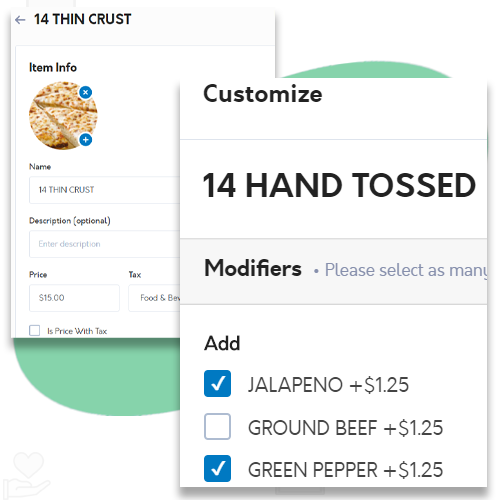The image features two overlapping partial screenshots on a white background with green circles. The first screenshot predominantly displays a user interface with a white background and black font. At the top-left corner, a gray back arrow is visible. Below that, "14 Thin Crust" is prominently labeled alongside "Item Info," accompanied by an image of a plain cheese pizza. Two blue circles are located beside the pizza image, one with an 'X' and the other with a '+' sign.

Further down, several text fields are labeled. The first field reads "Name: 14 Thin Crust." The next label states "Description (optional)" with an input field below prompting "Enter description." Following this, the fields show "Price: 15," "Tax: Food and Beverage," alongside a checkbox labeled "Is price with tax" which remains unchecked.

The second overlaid screenshot, positioned slightly to the right, also features a white background with black font. It is headed with "Customize: 14 Hand Toss," followed by a section labeled "Modifiers: Please select as many." Listed below are various topping options, each with associated prices. The first option, "Jalapeno," is checked for $1.25, marked by a blue box with a white checkmark. Below, "Ground Beef" priced at $1.25 is presently unchecked, in a plain white box. The last visible option is "Green Pepper," which is checked and indicated with a blue box and a white checkmark, costing an additional $1.25. 

The image is of excellent visual quality, featuring bold, easy-to-read text, and no other notable details.